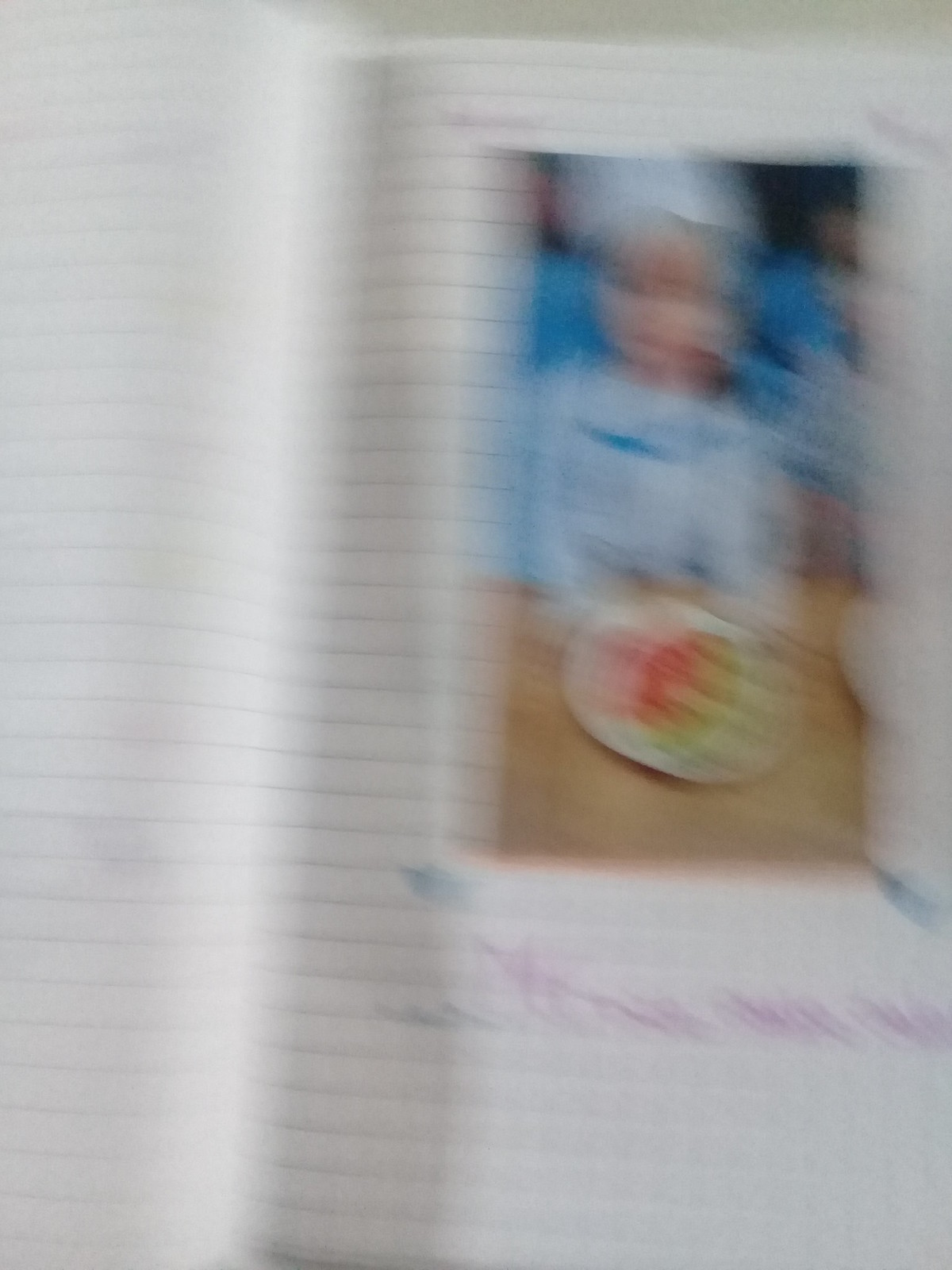A significantly blurred photograph depicts another photo placed on what appears to be an open notebook. The notebook's pages seem to have faint lines, which on closer inspection, might actually be very indistinct lettering, though it remains illegible due to the blurriness. Below the photo, a message penned in purple ink is visible; the writing is unusually slanted backwards, contrasting with the typical rightward slant of cursive handwriting.

The photo itself is a close-up of a child sitting at a tan table with a circular plate in front. The plate seems to hold a pink and green object, possibly a slice of watermelon. The child, whose features are obscured by the blurriness, might be in a hospital setting, inferred from a white covering on their head and what seems to resemble a hospital robe. There appears to be a medium blue pillow behind the child, whose skin looks fair. Due to the blurriness, further specifics are difficult to discern.